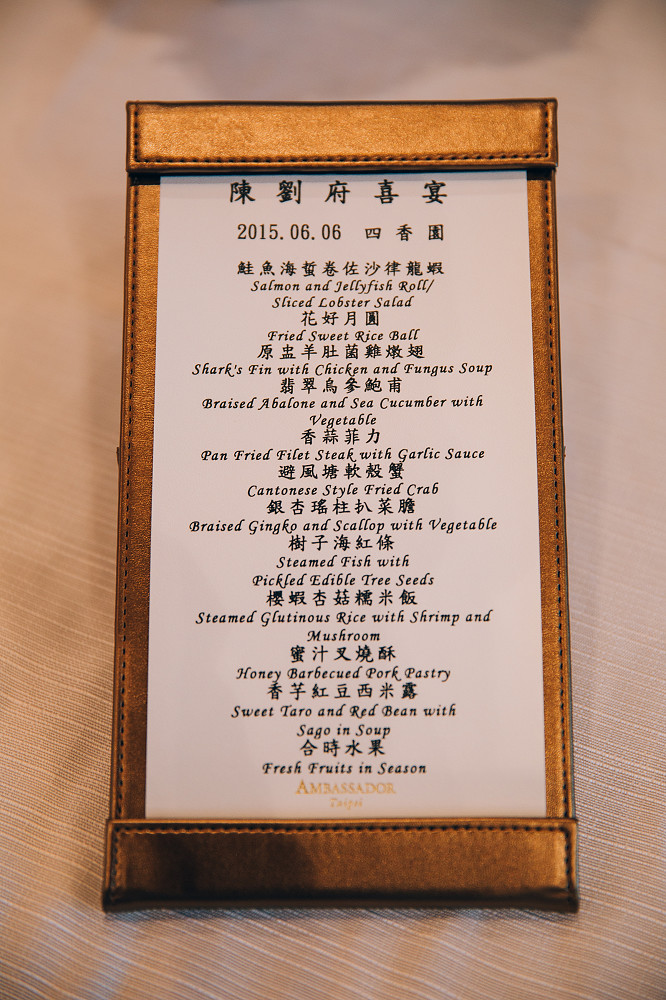The image showcases a detailed menu from a Chinese restaurant, presented in a sleek black leather cover with a white menu featuring black text at its center. The menu includes both Chinese characters and their English translations, listing a variety of dishes. It starts with the date "2015-06-06" and proceeds with items like salmon and jellyfish roll, sliced lobster salad, fried sweet rice ball, shark's fin with chicken and fungus soup, braised abalone and sea cucumber with vegetables, pan-fried filet steak with garlic sauce, Cantonese-style fried crab, braised ginkgo and scallop with vegetables, steamed fish with pickled edible tree seeds, steamed glutinous rice with shrimp and mushrooms, honey-barbecued pork pastries, sweet taro and red bean sago in soup, and fresh fruits in season. The menu is centered in the image, taking up the middle two-thirds, with the gray table forming the backdrop.